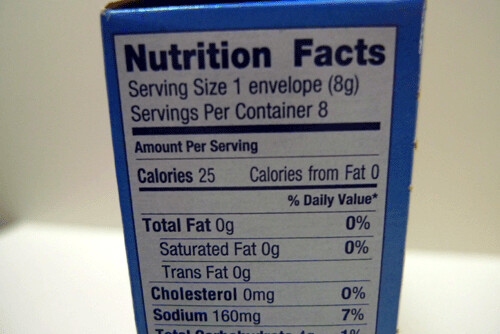The photograph features the nutritional information panel on the side of a box set against a plain white wall and a matching white countertop. The box has a distinct blue border framing the nutrition facts. The text is printed in a simple, legible black font on a white background, offering a clear contrast for easy readability. The nutrition facts indicate that each serving is one envelope, weighing eight grams, with a total of eight servings per container. Each serving contains 25 calories, with none of these calories derived from fat. The detailed breakdown lists the following per serving: total fat at 0 grams (0% of daily value), saturated fat at 0 grams (0%), trans fat at 0 grams, cholesterol at 0 milligrams (0%), and sodium at 160 milligrams (7%). The panel is partially cut off at the bottom, revealing only the top portion of the total carbohydrates section, where the percentage value is visible and indicated as a double-digit number, although the exact digits and gram amounts are obscured.